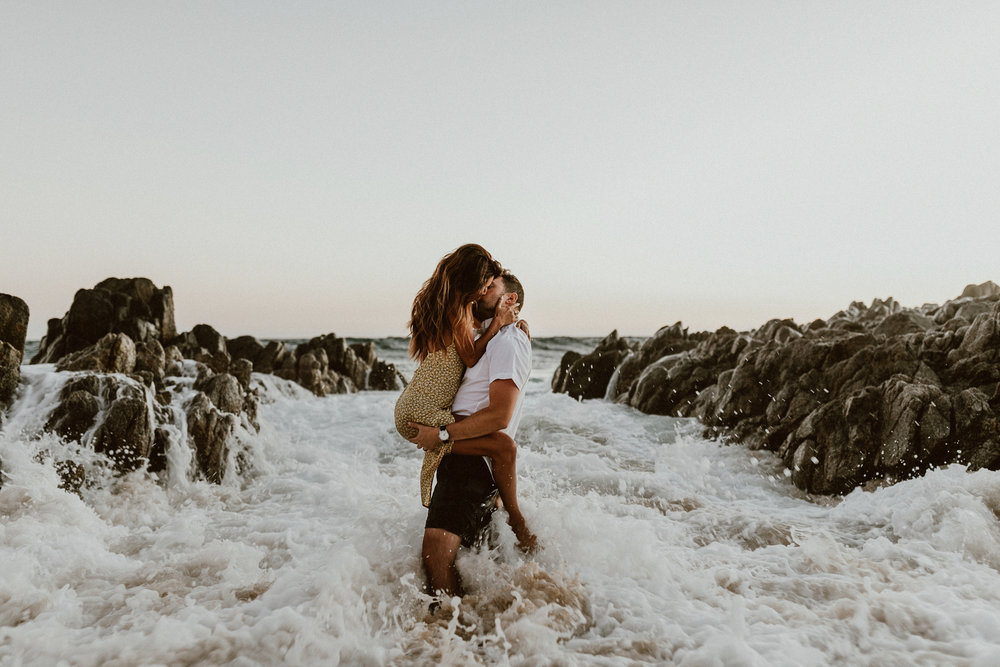In this photograph, a couple stands amidst the dramatic backdrop of rough ocean surf and surrounding rocks. The man, wearing a white t-shirt and either brown shorts or a bathing suit, braces himself against the crashing waves as he holds the woman tightly against his chest. Her long brown hair cascades down as she wraps her legs around his waist and kisses him passionately. She is dressed in a beige short dress, her feet just skimming the frothy tips of the waves. They are positioned slightly to the left of the center of the image, surrounded by large rocks on either side that rise four to five feet high. The ocean extends behind them with sizable waves rolling in. Overhead, the sky is a solid, cloudy gray, enhancing the romantic and dramatic ambiance of the scene.